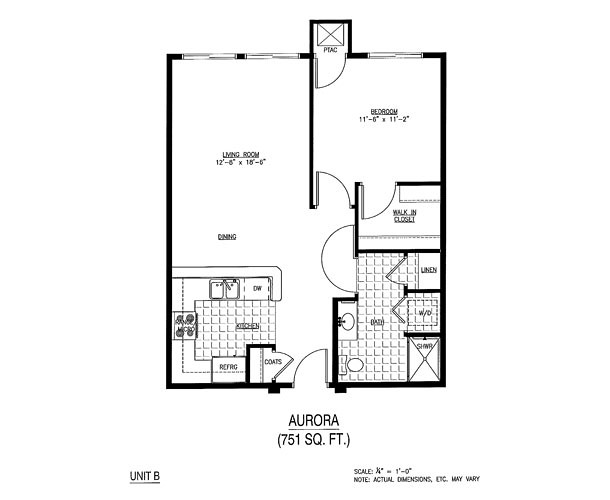This detailed floor plan depicts Unit B, known as the "Aurora," encompassing an area of 751 square feet. Rendered in a monochromatic color scheme, the layout provides a clear visual representation of the apartment's structure and dimensions.

In the bottom left-hand corner, the designation of the unit is clearly indicated. The right-hand section of the floor plan houses the bedroom, which measures 11 feet 8 inches by 11 feet 11 inches. Adjacent to the bedroom is a doorway leading into a spacious living room, sized at 12 feet 5 inches by 16 feet 8 inches.

Below the living room is the kitchen area, which includes designated spaces for essential appliances such as a refrigerator, sink, and oven. To the left of the kitchen is an expansive wall, which further defines the area.

The bedroom features a large walk-in closet located in the upper right-hand corner, providing ample storage space. Adjacent to the kitchen, on the right side, is the bathroom. The bathroom layout includes a toilet, a sink, a linen closet, and a shower.

Overall, the floor plan is well-organized, ensuring functionality and ease of movement throughout the Aurora unit.